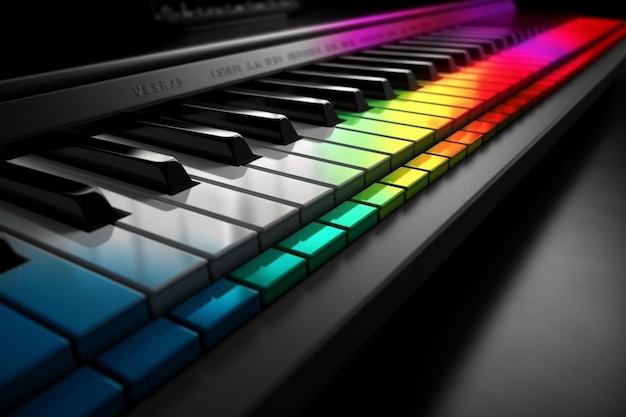The image shows a close-up side view of a large piano keyboard bathed in various colored lights. The piano has two layers of keys: the regular black and white keys on top, and an additional layer with parts of the white keys below. The body and the ground where the piano is placed are both gray. The keyboard is illuminated by rainbow-colored lights, creating a vibrant display across the keys. From left to right, the keys are tinted in shades of blue, white, green, yellow, orange, red, purple, and back to red. The piano also has some writing above the keys, which includes various letters and numbers like "B," "A," "S," and "6," although some of the other text is unclear due to the image quality. The captivating lighting adds a dynamic and colorful texture to the image, highlighting the intricate details of the piano.